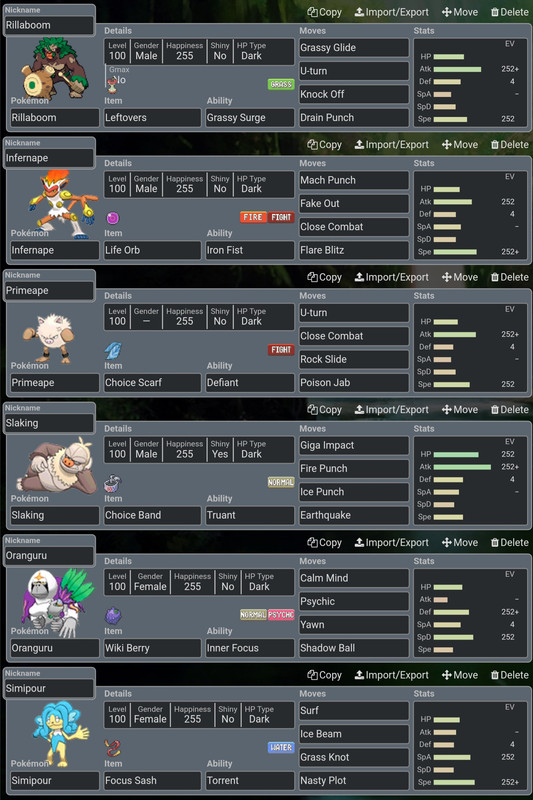The image depicts a comprehensive stats page featuring six Pokémon characters, each presented in a detailed horizontal section. The characters included are Rillaboom, Infernape, Primeape, Slaking, Oranguru, and Simipour. Each character's section begins with a cartoonish illustration of the Pokémon, positioned just below their respective names. Adjacent to the names are details such as the Pokémon's level, gender, happiness level, shiny status, and hit points (HP) type.

Beneath these details, the item and ability associated with each Pokémon are listed. For example, Rillaboom uses the item Leftovers and has the ability Grassy Surge. Moving further right, each Pokémon's moveset comprising four moves is provided. Rillaboom's moves include Grassy Glide, U-Turn, Knock Off, and Drain Punch, while Infernape's moves are Mach Punch, Fake Out, Close Combat, and Flare Blitz.

On the far right of each section, the specific stats for each Pokémon are displayed. These stats encompass attributes such as HP (Hit Points), ATK (Attack), DEF (Defense), SPA (Special Attack), SPD (Special Defense), and SPE (Speed).

Overall, this thorough layout offers a detailed snapshot of each Pokémon's attributes, abilities, and combat moves.